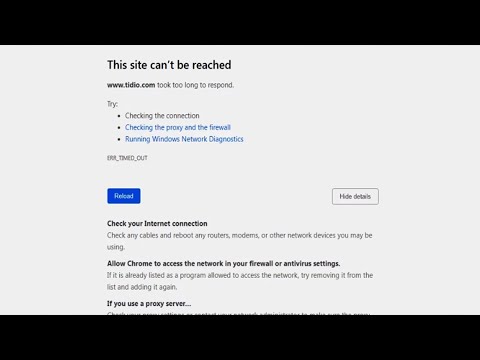In this image, a screenshot captures a desktop screen displaying a website experiencing a network failure. The webpage features distinct elements for clarity:

- The top and bottom of the screenshot are bordered in black.
- The main area of the image has a light gray background.
- Prominently displayed in the center is a message reading "This site can't be reached," written in black text.
- Below the main text, the URL "www.tdio.com" is mentioned, also in black text, alongside a note: "100k, it took too long to respond."
- Suggestions for troubleshooting are listed, including:
  - "Try checking the connection," in black text.
  - "Checking the proxy and the firewall," and "Running Windows Network Diagnostics," both in blue text.
- At the bottom, errors are summarized with "ERR_TIMED_OUT" in black text.
- There is a rectangular button labeled "Reload" with white text on a blue background.
- Another option, "Hide details," is written in black text.
- Additional troubleshooting steps appear in bold black text:
  - "Check your internet connection."
  - "Allow Chrome to access the network in your firewall or antivirus settings."

The overall layout is clean and straightforward, ensuring the error and potential solutions are easy to read and comprehend.